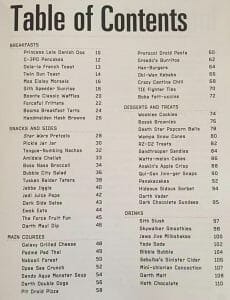This image captures a table of contents page from what appears to be a recipe book. The text is too small to be legible, but the layout suggests various sections typically found in culinary guides. The first heading likely lists "Breakfast" options, followed by a section possibly titled "Sides" or "Sides and Salads." Subsequent headings seem to include "Soups and Sides" or "Salads and Sides," then "Main Courses." Another section appears to cover "Desserts," perhaps specified further as either "Desserts and Treats" or "Desserts and Fruits." The final section is assumed to be for "Drinks." The table of contents page is the sole focus of this image, with no additional content visible.